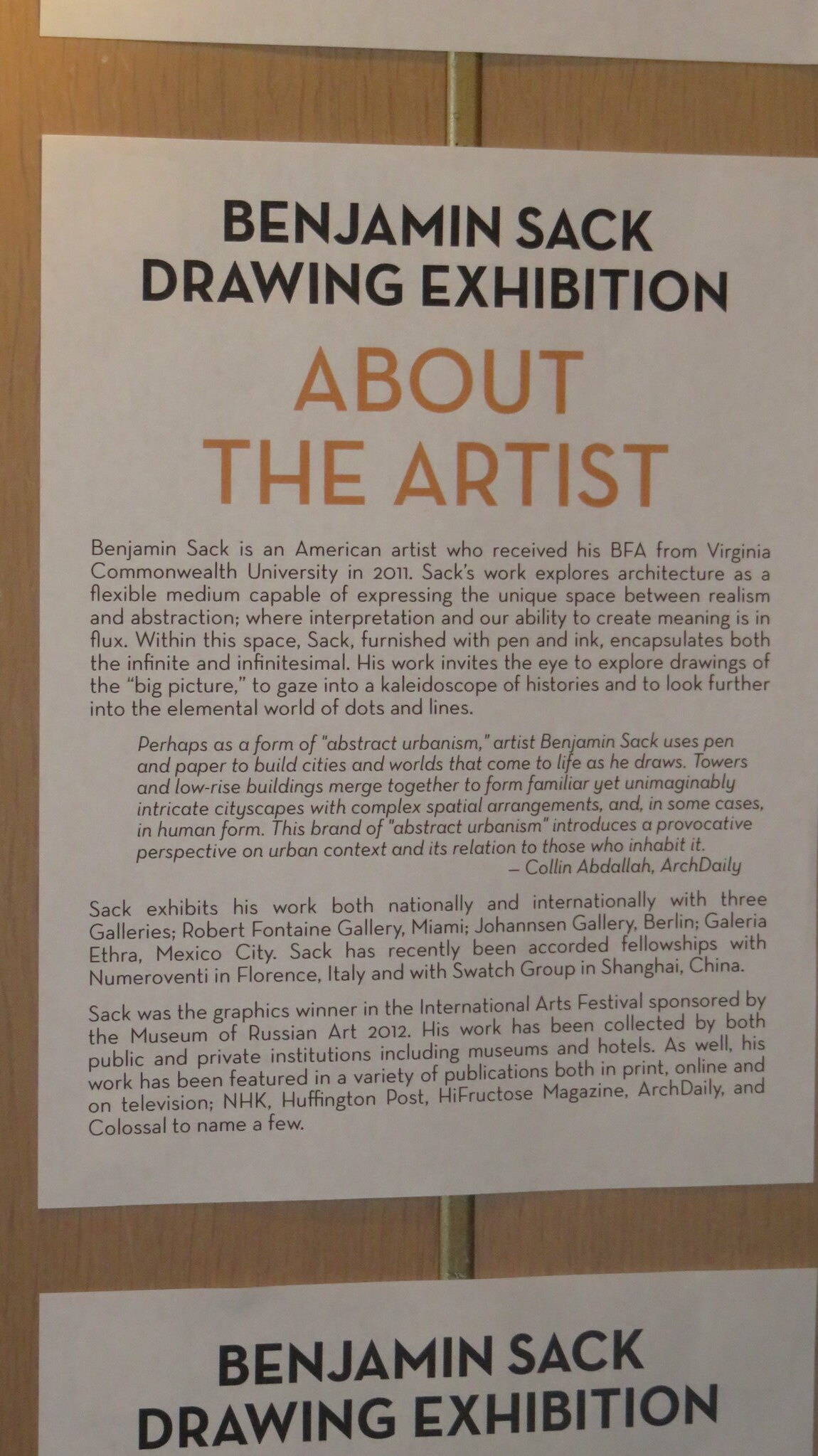The photograph depicts a wooden wall with a metal stripe running vertically down the center. Several pieces of paper are posted on the wall, all related to artist Benjamin Sack. The main visible paper, printed on white with black lettering, prominently features the title "Benjamin Sack Drawing Exhibition" at the top. Below the title, in larger orange letters, it reads "About the Artist." The detailed text beneath begins with, "Benjamin Sack is an American artist who received his BFA from Virginia Commonwealth University in 2011." It goes on to elaborate on Sack's artistic focus, noting that his work explores architecture as a flexible medium. The description continues with an analysis of his style, stating, "His work invites the eye to explore drawings of the big picture to give into a kaleidoscope of histories into the elemental world of dots and lines." At the bottom of the main page, some text is too small to discern clearly. Below this sheet, another similar page is partly visible, hinting at more information or possibly a repetition of the title "Benjamin Sack Drawing Exhibition."